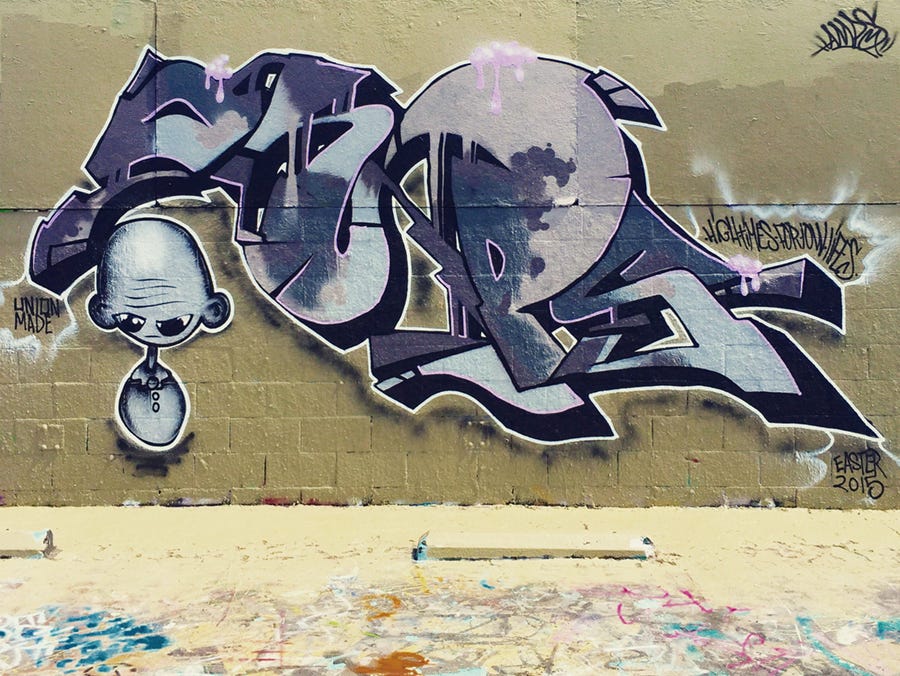The image features a vibrant graffiti tag prominently displaying the phrase "Linden Maid" at one end, with "Linden Maid" highlighted in white trailing off the letters, which are depicted in a striking black. The mural is a masterpiece of urban art, painted in an array of purple, gray, light gray, white, and black hues, creating a metallic sheen through expert use of shading and paint type.

In the midst of the intricate design, an indecipherable "P" stands out, surrounded by nearly unreadable winding arrows. Drops of pink drip from the top of the letters, adding a dynamic element to the piece. On the same tan concrete wall, there's a striking black and white (or light gray) depiction of a person with a bald head and sticking out small ears. This figure, with its large eyes, thin neck, and oval-shaped head, sports a buttoned-down polo shirt with a collar but notably lacks arms. The artist has outlined the person in white, seamlessly integrating the character with the surrounding letters, adding a fascinating layer to this enigmatic graffiti.